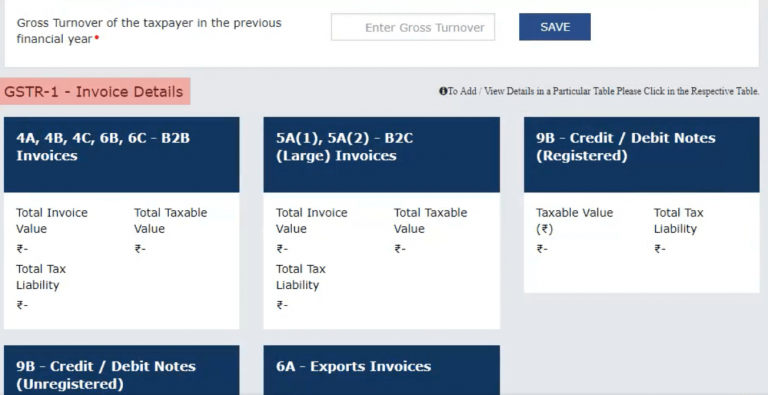This image depicts a digital invoice section for a business, featuring an interface with various informational and input fields. The entire page has a light gray background, providing a neutral and professional appearance.

At the very top of the page, there is a prominent white box labeled "Gross turnover of the taxpayer in the previous financial year." Adjacent to this label is an empty input box, followed by a "Save" button towards the far right.

Beneath this top section, on the left side, the page displays a title that reads "GSTR-1 Invoice Details." To the right of this title, an instructional note indicates, "To add/view details in a particular table, please click in the respective table."

The interface further breaks down into three main sections. On the left, there is a box for "Invoices"; in the center, a box for "Large Invoices"; and on the right, a section for "Registered Credit and Debit Notes." At the bottom of the page, there is an additional section labeled "Unregistered Debit and Credit Notes" alongside "Exports Invoices."

The layout clearly organizes the different types of financial records, facilitating easy navigation and data entry for business users managing their invoicing and tax details.